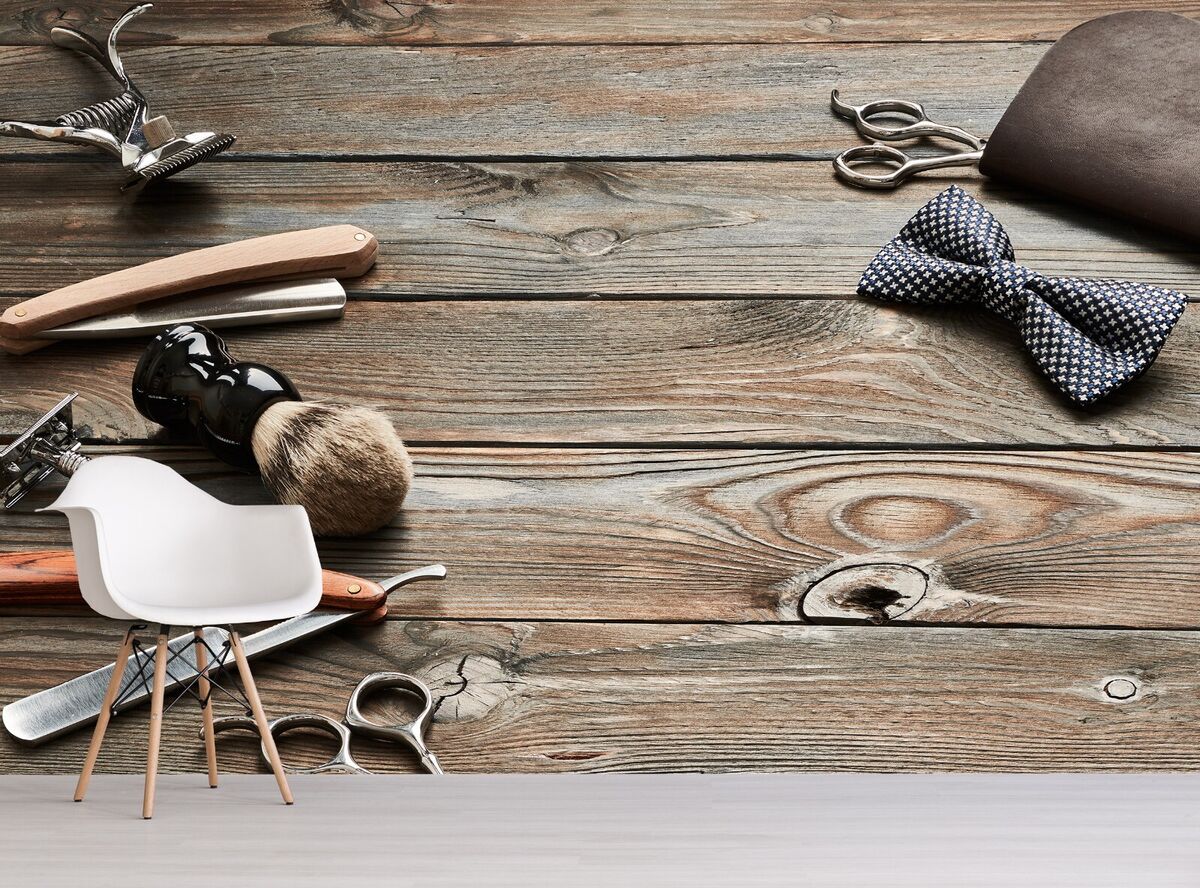The image showcases a rustic barbershop and beauty arrangement set against a backdrop of dark brown, weathered wooden planks, detailed with visible aging lines. The wooden background is adorned with various grooming tools, including a pair of silver scissors, a straight razor with a brown handle, a metal razor, a manual clipper with handles you squeeze together, and a shaving brush commonly used for applying shaving cream. Also featured is a blue and white polka-dotted bowtie, a leather strap, and a leather case with a pair of metal scissors protruding out. The scene extends onto a gray floor where a white plastic chair with brown wooden legs is positioned, adding a tactile, real-world element to the otherwise photographic depiction of grooming elegance captured in the detailed wooden background.